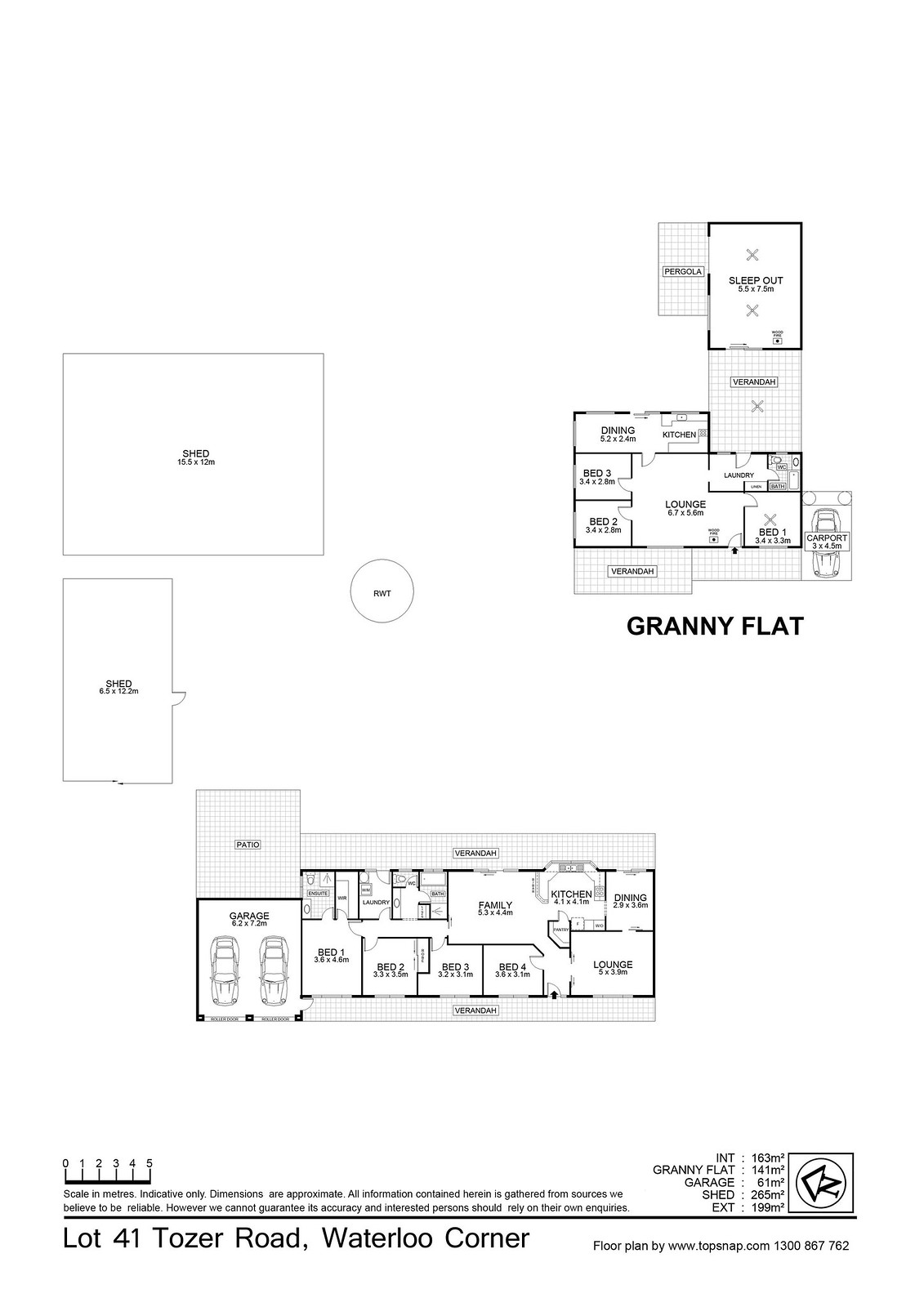The image features a series of detailed diagrams, each with annotations in fine print. In the top left corner, there is a square diagram with small, black text in the center. Beneath this, to the left, lies a rectangular diagram with similar small writing, and an open section on the right side that resembles a door. Adjacent to these, on the right, is a small circular diagram, again with fine text.

Above and to the right, a label reads "Granny Flat." This section displays another diagram, illustrating various rooms, some of which are shaded. All rooms contain very small black writing, making it difficult to read. At the bottom of the page, there is another detailed diagram featuring what appears to be a two-car garage along with several rooms, some of which are also shaded.

At the very bottom, in black text, the diagram is labeled "Lot 41 Tozer Road Waterloo Corner." It also includes a note indicating it is a "Floor plan by www," though the remaining letters are too small to discern. Above this, there is a scale with explanatory text that is also small and somewhat out of focus. To the right, a key explains the different shadings used in the diagrams, but this text is also very small.